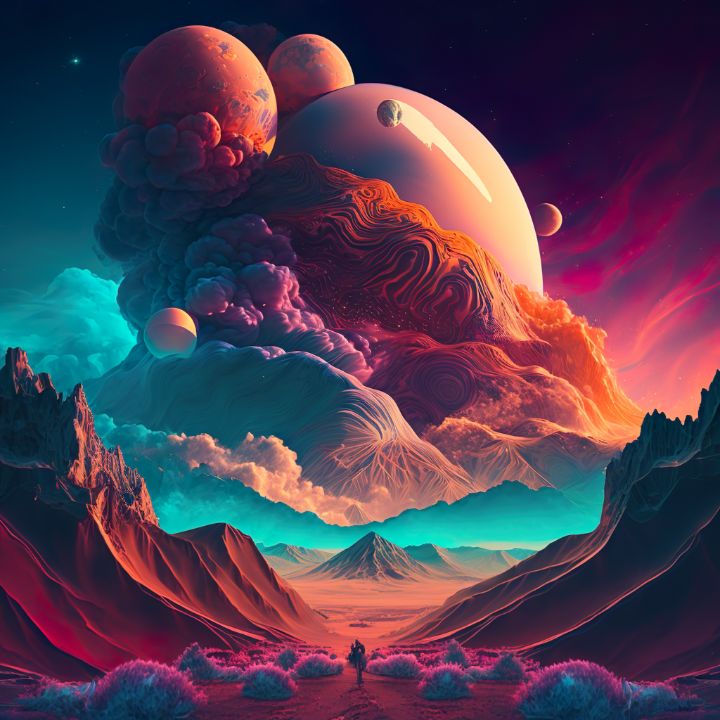This is a highly detailed, computer-generated or AI-created fantasy image of an otherworldly scene in outer space. The landscape features a valley surrounded by craggy, steep mountains that come in vibrant colors like magenta, pink, orange, teal blue, aquamarine, red, and maroon. The ground appears to have purple mountains and slopes with stretches of desert in contrasting shades of pink, purple, and orange. In the middle of this surreal scene, there is either a small figure or a tree, adding a focal point amidst the alien terrain.

Above this colorful landscape is a mesmerizing, abstract sky. It is a riot of swirling colors and textures, with different planets and cosmic gases superimposed in a dreamlike fashion. The sky displays blends of magenta, pink, orange, and teal blue, and includes an aqua-colored section filled with rolling, smoke-like forms. On one side of the sky, a large, circular planet is visible with at least four smaller planets converging around it, further adding to the fantastical quality of the image. There's also a purple sky segment featuring a planet, alongside a blue sky with a small star in the far left corner.

Overall, the image is an artistic and abstract portrayal of what space might hold, filled with vibrant colors, varied terrains, and celestial bodies that inspire wonder and imagination.